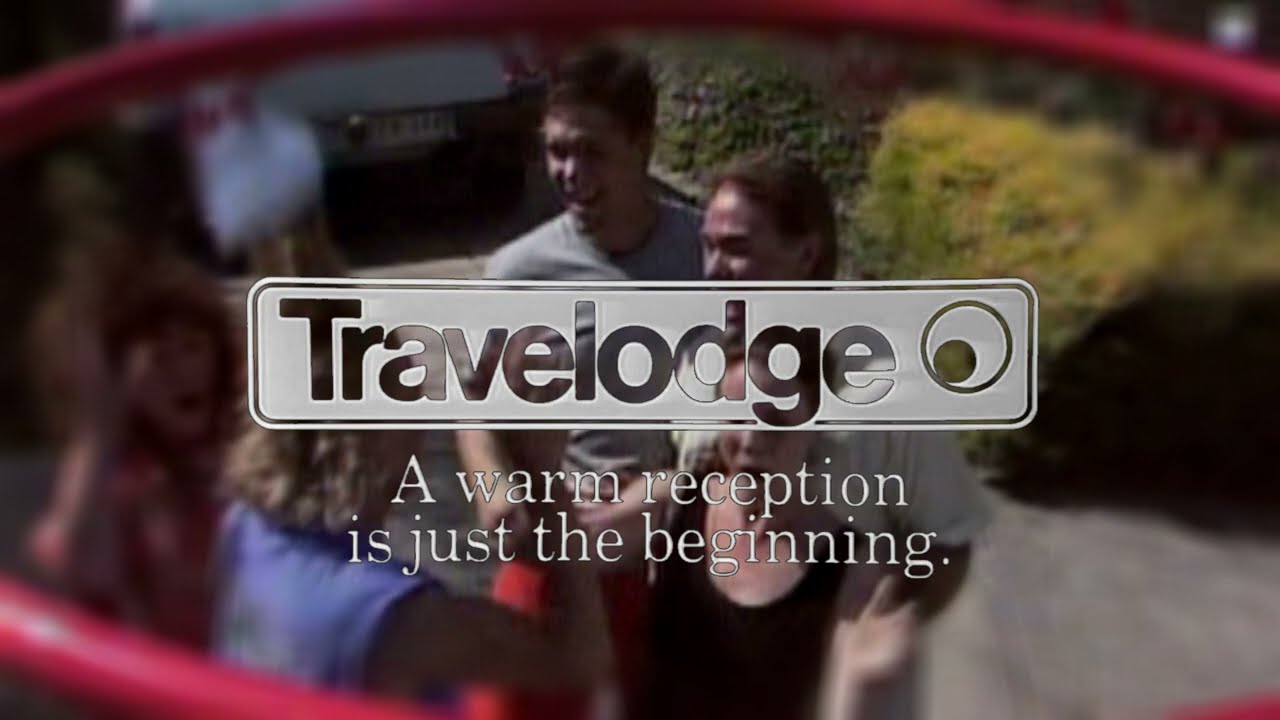The image is an advertisement for Travelodge, prominently displaying the Travelodge logo within a gray rectangular box that features transparent lettering. Below the logo, in silver and white text, it reads, "A warm reception is just the beginning." The scene, as viewed through a red-rimmed oval border resembling the edge of a basketball hoop, captures a group of five people—three women and one man on the left, and two women on the right—all engaged in animated conversation. The background is intentionally blurred but suggests an outdoor setting, featuring a sidewalk, some bushes, a partially visible vehicle with a license plate, and bright, sunny conditions. The advertisement focuses on the theme of welcoming and friendly service, as highlighted by the central, clear text and logo.